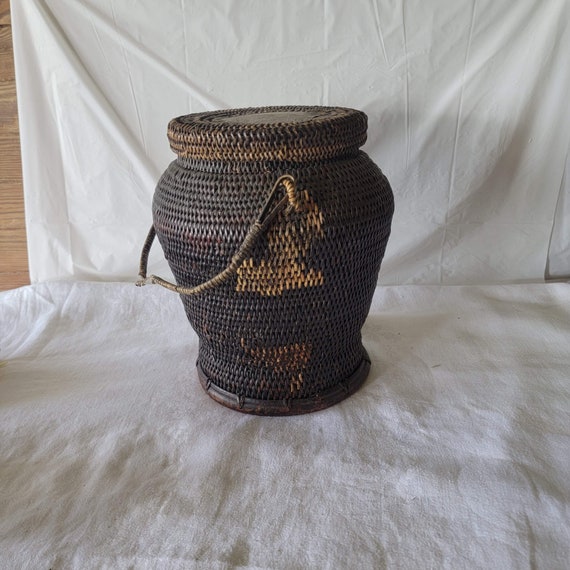A color photograph features an old, urn-shaped wicker basket with a tight, dark brown weave, accented by lighter patches and a lighter-colored broken handle. The basket, which resembles those used by traditional snake charmers, also has a lid and exhibits signs of wear, likely from age and possible insect damage. The scene is set against a backdrop of a draped white cloth, with another white sheet on the floor, partially revealing light wooden wall paneling. Shadows from the basket cast a gray hue onto the white sheets, adding depth to the vintage aesthetic.